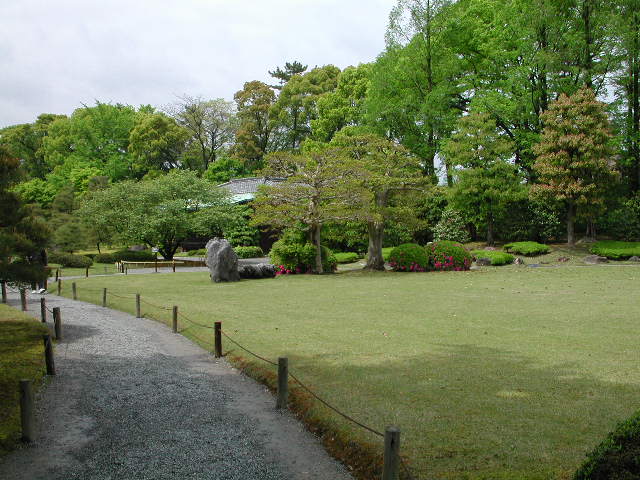The photograph captures a beautifully manicured park or garden during the daytime. Dominating the scene in the lower left-hand corner is a gravel pathway bordered by wooden posts and a single line of rope forming a rustic barrier. This pathway cuts through lush, recently mowed green grass that extends to the right. Along the midline of the image, delineating the transition from grass to more cultivated garden areas, is a charming row of azalea bushes adorned with pink flowers. Various ornamental trees, some with flattened, bonsai-like forms, rise up from this line, increasing in height from left to right until they reach the top of the frame. The leaves of these trees exhibit a spectrum of colors, including green, whitish, reddish hues, and their branches are intermingled with smaller shrubs. Among the foliage, a couple of stones add texture and interest. Partially concealed in the upper left-hand corner beneath these trees, the light-colored roof of a building peeks out. Above, the sky is a mix of light blue and gray with scattered clouds, enhancing the serene atmosphere of this meticulously maintained outdoor space.